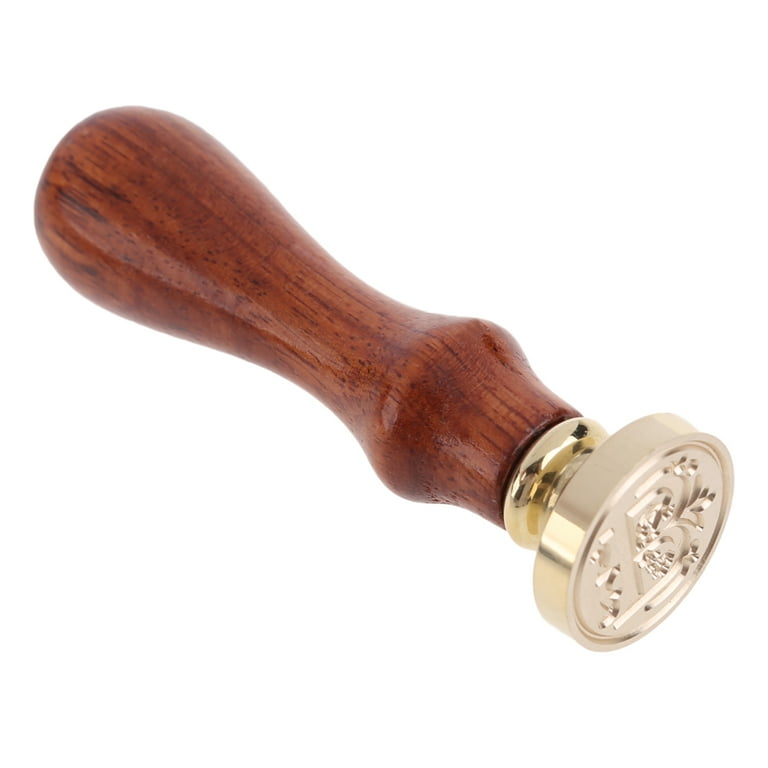This detailed photograph showcases a close-up view of a traditional wooden-handled stamp set against a pristine white background. The stamp's head, situated prominently at the bottom right corner of the image, is circular in shape and crafted from a glossy, golden metal. This reflective metal head, adorned with intricate designs surrounding a central 'B' shape, captures light along its rim where it joins the handle. The ergonomic wooden handle, made from medium brown-stained wood, features a lathe-turned design: it curves gracefully outward, dips inward at the center, and expands into a bulbous top, providing an easy grip. The image is devoid of any other colors or textures, emphasizing the fine details of the stamp and handle alone.